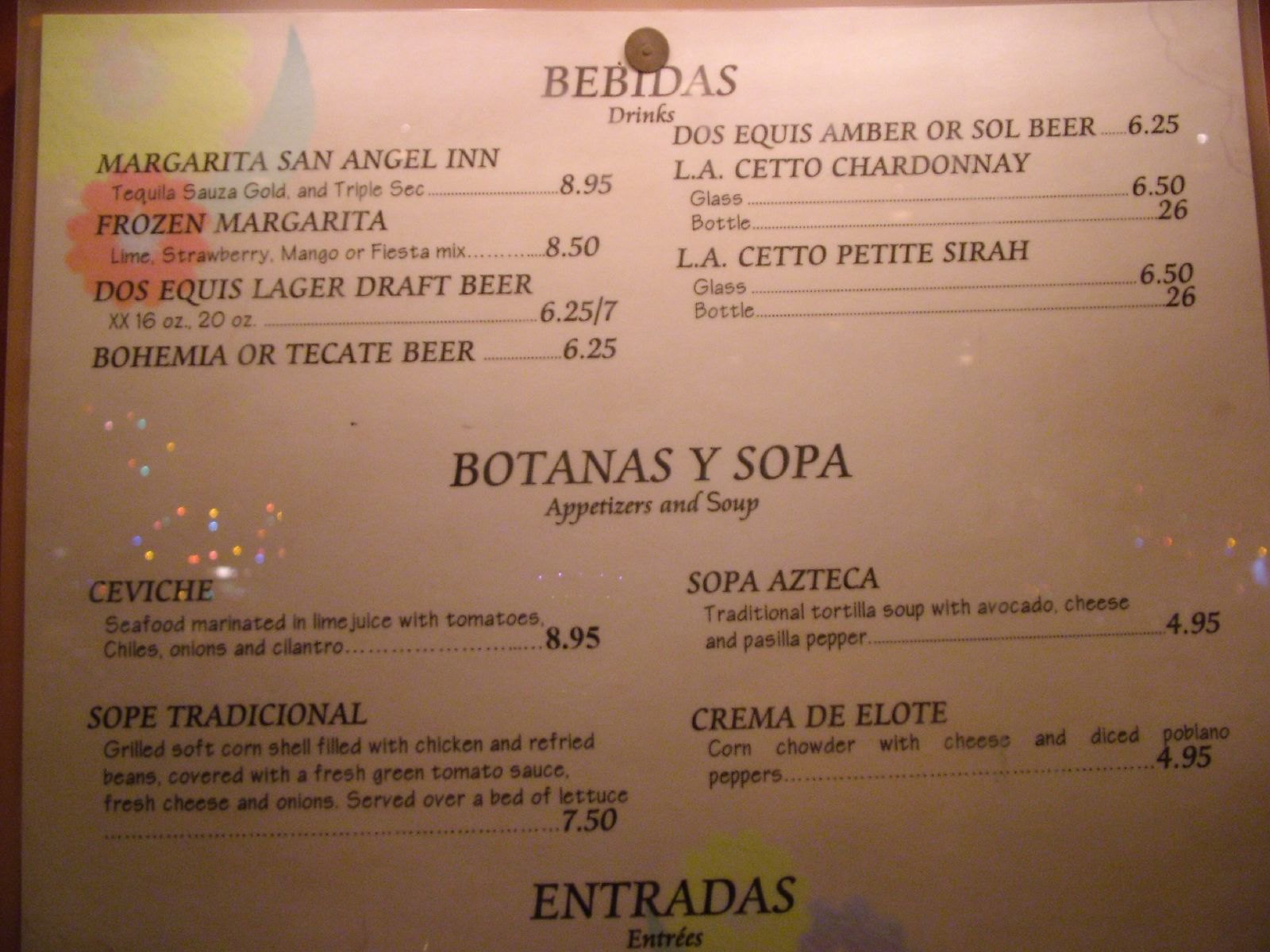The image is a cropped picture of a menu featuring a goldish border visible on the left side and slightly in the upper right corner. The menu's backdrop is a whitish color. At the top-center of the menu is a brown pin, below which is a Spanish phrase followed by the word "Drinks." The drinks section lists six different alcoholic beverages, each with its English translation indicating their ingredients. Beneath the drinks section are the "Appetizers and Soup," consisting of four items, each with English descriptions and their respective prices. The bottom section, presumably the entrees, is cut off in the image. In the upper left corner of the menu, there are two flowers; a larger yellow flower above a smaller red one. Additionally, a yellow flower marks the entrees section.